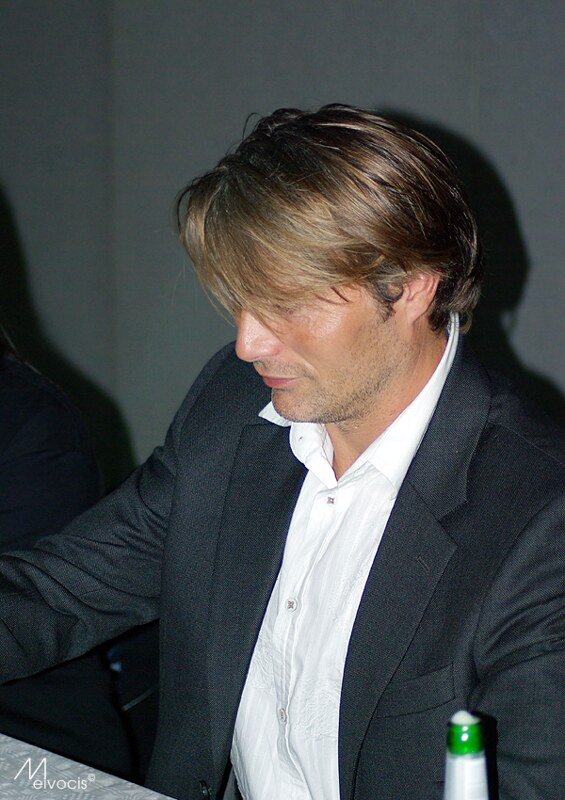A dimly lit scene captures a man seated at a table, facing slightly to the left. His medium-length, dirty blonde hair, streaked with grey, is combed to the side, and he sports a five o'clock shadow sprinkled with grey. The man is dressed in a black jacket over a white button-up, collared shirt. The photograph, taken from the right, showcases his contemplative demeanor as he gazes down at the table. Behind him, a shadowy, white wall forms the backdrop, further accentuated by a focused light illuminating him from the front. In the bottom right corner of the image, the top of an open green glass bottle is visible. Additionally, in the bottom left, a watermark reading "Melvocis" accompanied by a copyright symbol can be seen. The table surface appears to be textured metal. The combination of these elements creates a poignant and introspective atmosphere around the subject.